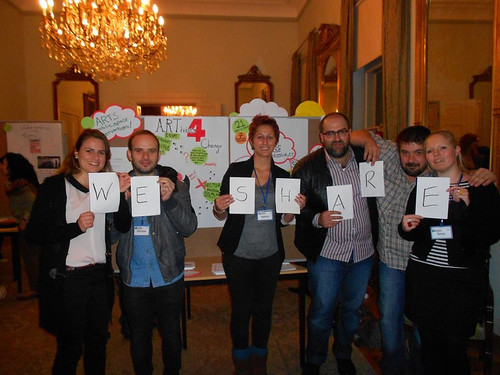The image depicts six individuals standing in a row at an indoor event, each holding up white sheets of paper that collectively spell out "WE SHARE." The group consists of three women and three men, each dressed in semi-formal attire and wearing lanyards, indicative of a work event or convention. From left to right, the first woman wears a black jacket and pants with a white shirt and holds the letter "W". The young man next to her, in a gray jacket, blue shirt, and black pants, holds the letter "E". The second woman, in a black jacket, gray shirt, and black pants, holds the letters "S" and "H". The middle-aged man beside her, dressed in blue jeans and a collared shirt with stripes, holds the letter "A". Another middle-aged man in jeans and a checkered collared shirt holds the letter "R". The last young woman, in a black jacket and black-and-white striped shirt with black pants, holds the letter "E".

Behind the row of people, there's a display board labeled "ART FOUR" adorned with various labels and posters, which further emphasizes the event's focus on art and collaboration. The room features soft yellow walls with brown-framed mirrors, enhancing the elegant ambiance created by a chandelier with glowy lighting hanging above. In the background, additional attendees and tables with project displays suggest a busy convention environment dedicated to sharing creative or work-related ideas.